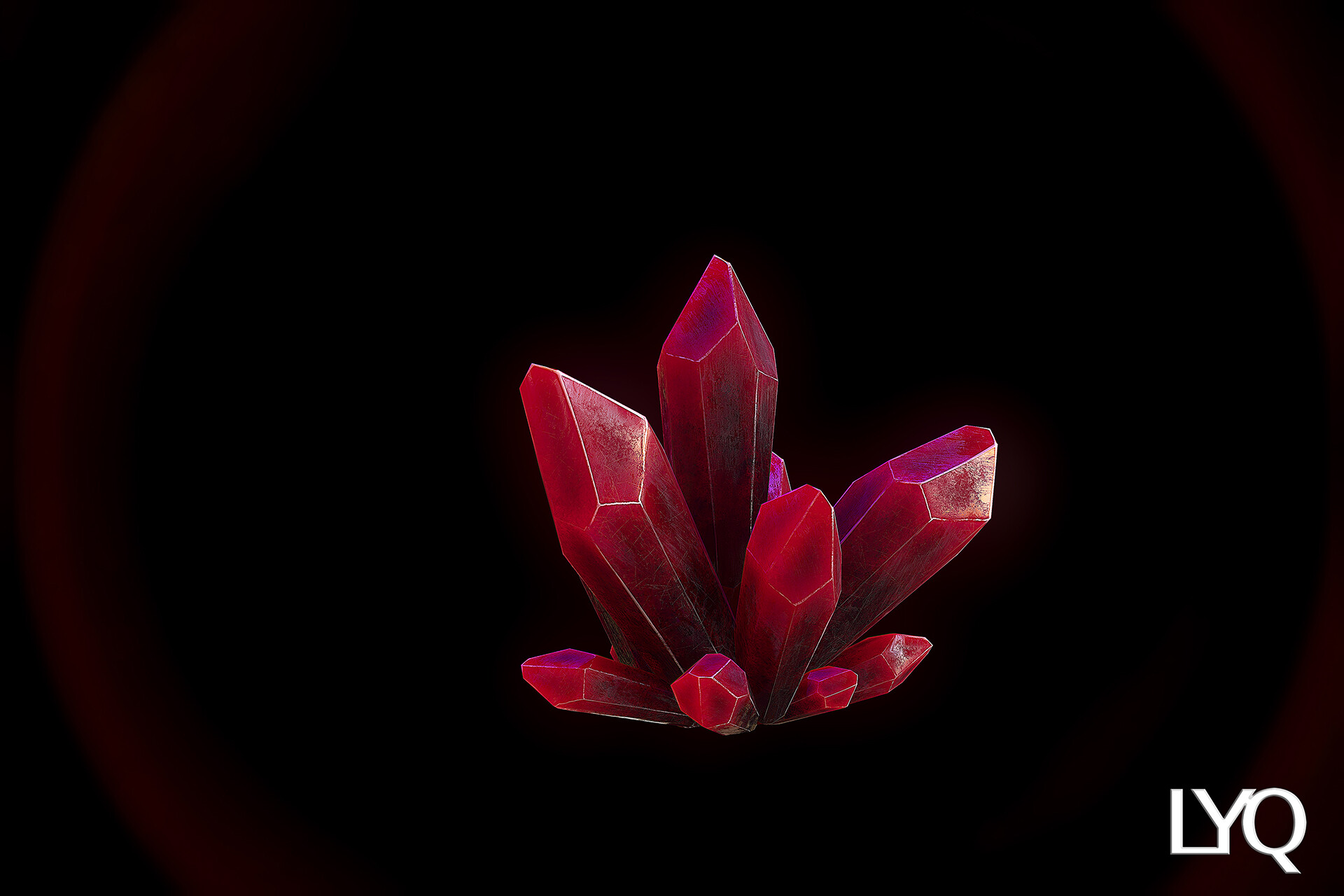The image is a rectangular photograph or a digitally created piece with a predominantly solid black background, subtly illuminated by a faint, almost indistinguishable red orb around the edges. In the bottom right corner, the white lettering "LYQ" is prominently displayed. At the center of the composition, a striking arrangement of reddish-pinkish-purplish crystals emanates outward, resembling an intricate, crystalline flower or an artistic sculpture. The central feature comprises a total of eight crystals: four larger ones reaching upwards and outwards, accompanied by four smaller ones forming a supportive base. The 3D effect of the crystals conveys a sense of depth and texture, enhancing the visual impact of the piece. The overall impression is of a meticulously crafted image where the vibrant hues of the crystals contrast starkly with the dark background, creating an eye-catching and mysterious visual experience.